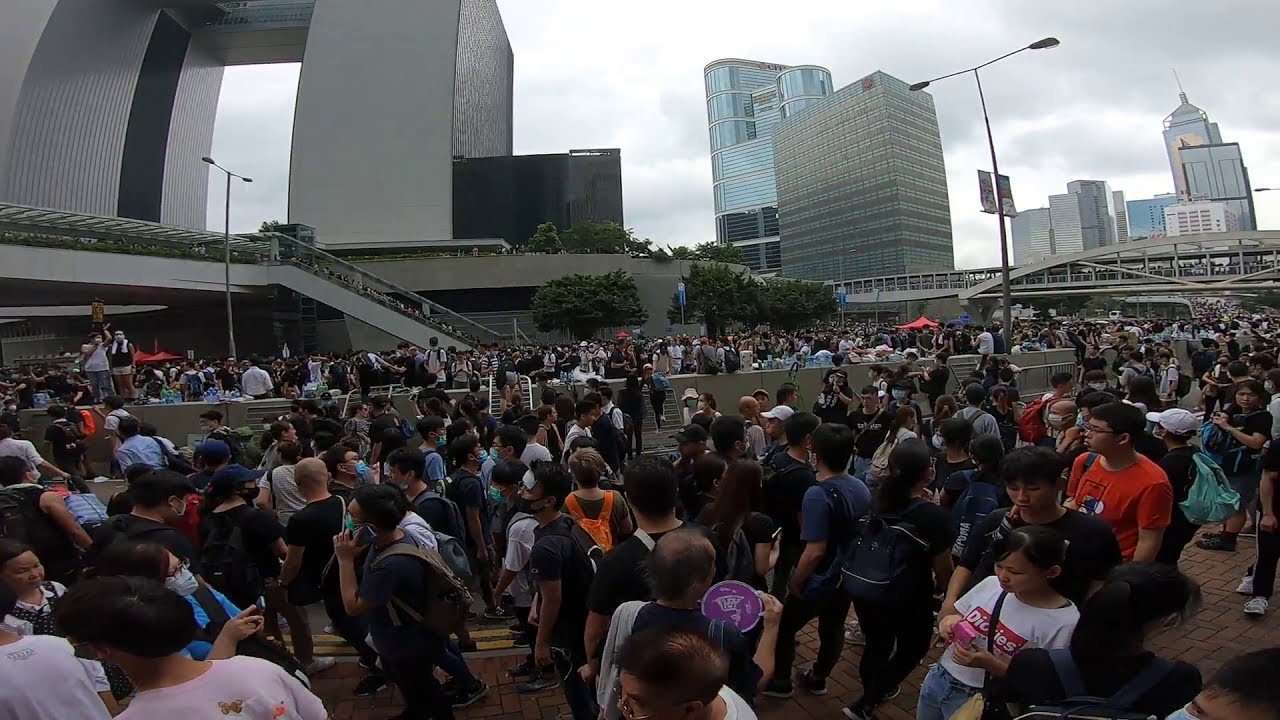In this photo, we see a bustling city scene characterized by a large crowd gathered in what appears to be a business district filled with tall skyscrapers and corporate buildings. The sky above is grey and cloudy, and several green-leafed trees dot the area, adding a touch of nature to the urban environment. Predominantly, the crowd seems to consist of Asian and Indian individuals, many of whom are carrying backpacks, suggesting they may be attending a convention or a large gathering. Concrete steps are visible in the distance, flanked by a concrete wall where some people are sitting. Prominently, there are two tall, glass office buildings side-by-side, with another cluster of high-rises to the right. A bridge teeming with people can be seen in the background, and two tall awnings provide shelter over the stairs leading into the crowd. Streetlights are interspersed throughout the scene, contributing to the cityscape ambiance.